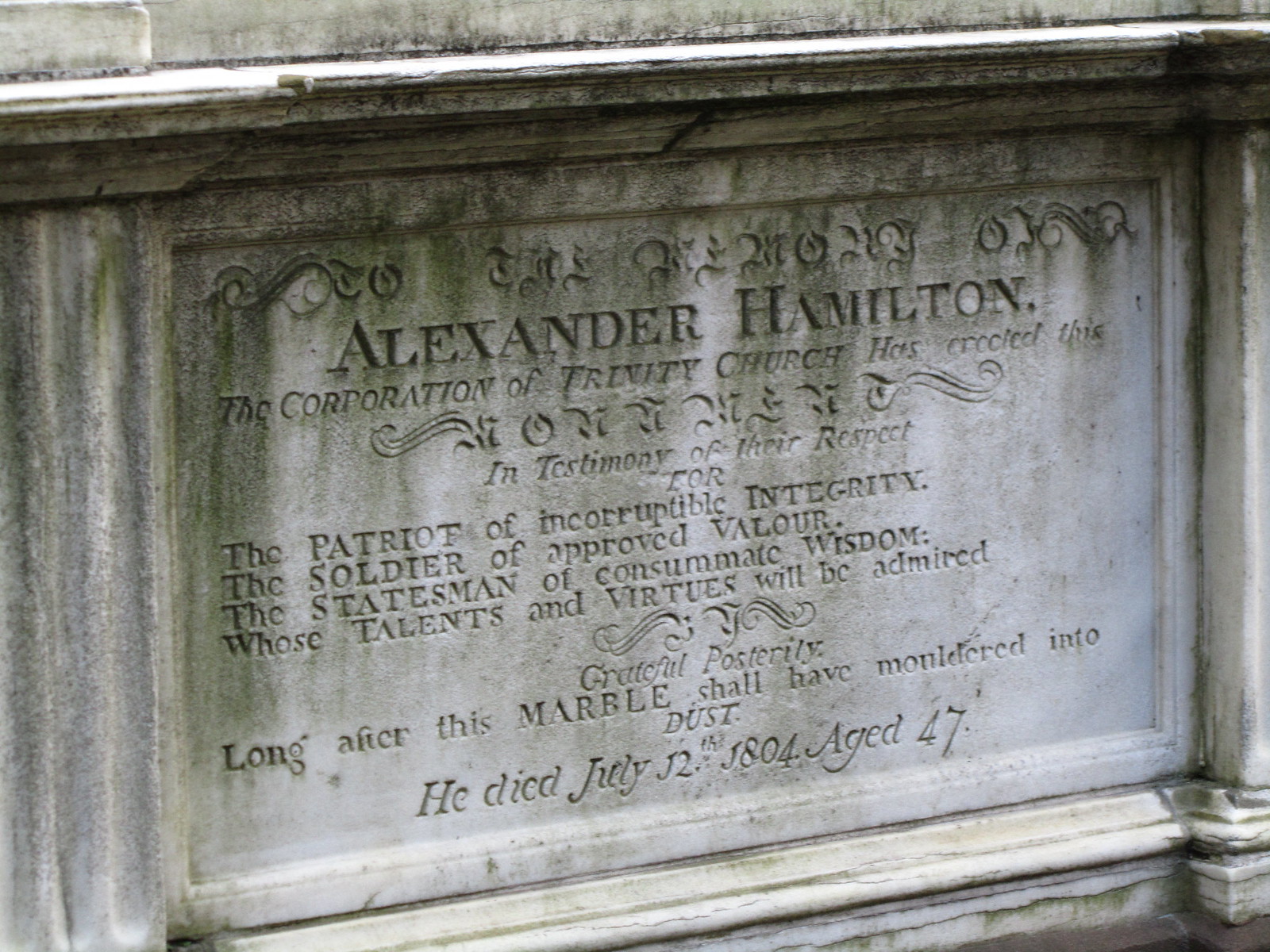The photograph captures a weather-worn grave marker of Alexander Hamilton, recipient of considerable respect from the Corporation of Trinity Church. The stone, seemingly marble, bears intricate detailing at the top and is significantly darkened and grimy due to age and mildew accumulation, particularly around the upper sections. The inscription, although somewhat obscured by the grime, reads:

- **Alexander Hamilton**
- "The Corporation of Trinity Church has erected this in testimony of their respect for the patriot of incorruptible integrity, the soldier of approved valor, the statesman of consummate wisdom, whose talents and virtues will be admired. Grateful posterity long after this marble shall have moldered into dust. He died July 12, 1804, aged 47."

The image is taken from a diagonal angle, causing the right side of the marker to recede into the distance, revealing areas where the stone appears slightly cleaner towards the bottom.